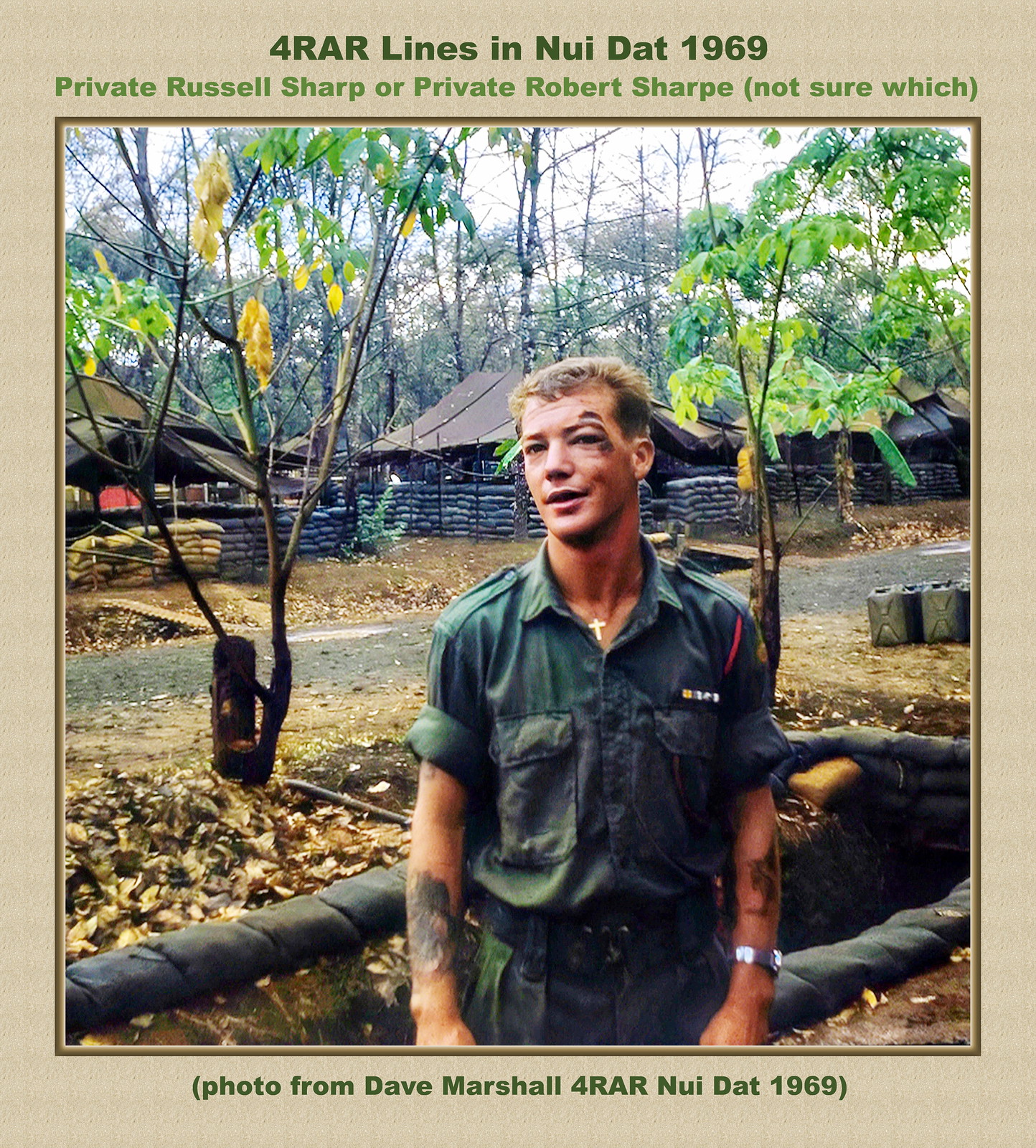This is an older full-color photograph taken in 1969 at Nwai Dat, showing a soldier outdoors in the daytime. He is wearing a green military uniform with the sleeves rolled up, showcasing tattoos on his arms. A cross necklace hangs around his neck. His left eye appears bruised as if he had been punched, marked by some noticeable black discoloration. The backdrop reveals a military base with multiple sandbagged bunker areas, wooden shelters, and numerous trees. The setting is dusty with patches of grass and foliage visible. The photograph, framed in brown, bears the inscription "4 R.A.R. 1969" and is credited to a photographer named Dave Marshall. Although the soldier is identified as Private Russell Sharp or Private Robert Sharp, there is uncertainty about which brother he is. The man stands confidently, possibly grinning, and is wearing a wristwatch, exuding a blend of toughness and resolve.